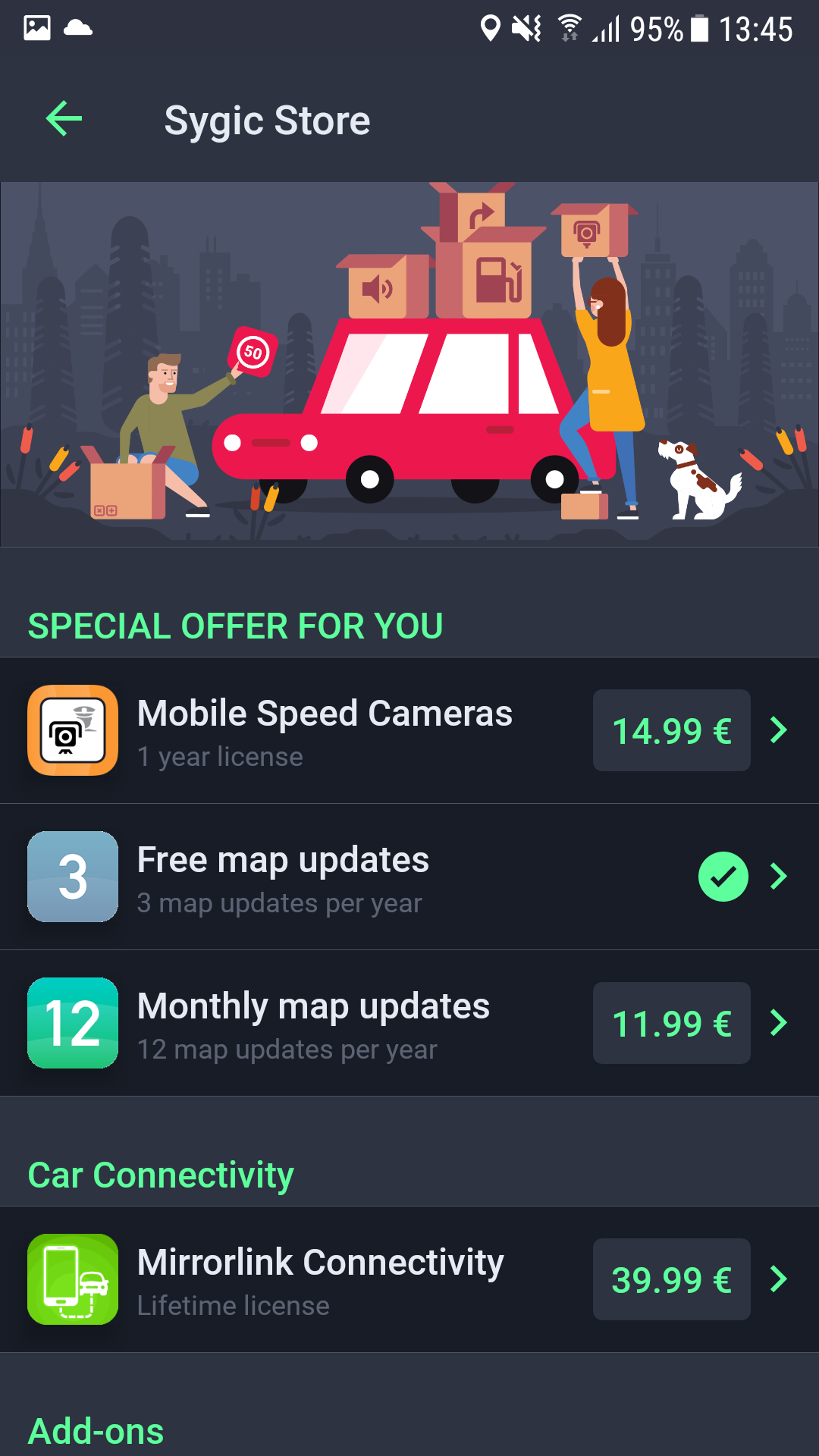The image features a screen resembling the size of a cell phone display, characterized by a black background. At the top, there's a green, left-facing arrow next to the text "CIGIC Store," with the "S" and "Store" capitalized. Below this header is a section displaying an illustration of two people stacking boxes onto a red car. The man in the foreground holds a red square sign with the number "50" inside a circle, while the woman, beside him, places a box adorned with a camera icon. A dog stands at the woman's feet, observing the activity.

Further down, a green banner reads "Special Offer for You." Following this, a series of rectangular segments each contain right-facing arrows. The first segment displays a camera icon and the text "Mobile Speed Cameras," priced at $14.99. The second features a grayish-blue rectangle with the number "3" and reads "Free Map Updates," accompanied by a green circle with a black checkmark. The third segment highlights "Monthly Map Updates" inside a 12-marked yellowish-green square, priced at $11.99. The fourth and final segment mentions "Car Connectivity" in green, featuring a green mirror link icon and a price of $39.99. At the screen's bottom left corner, there's a green label reading "Add-Ons."